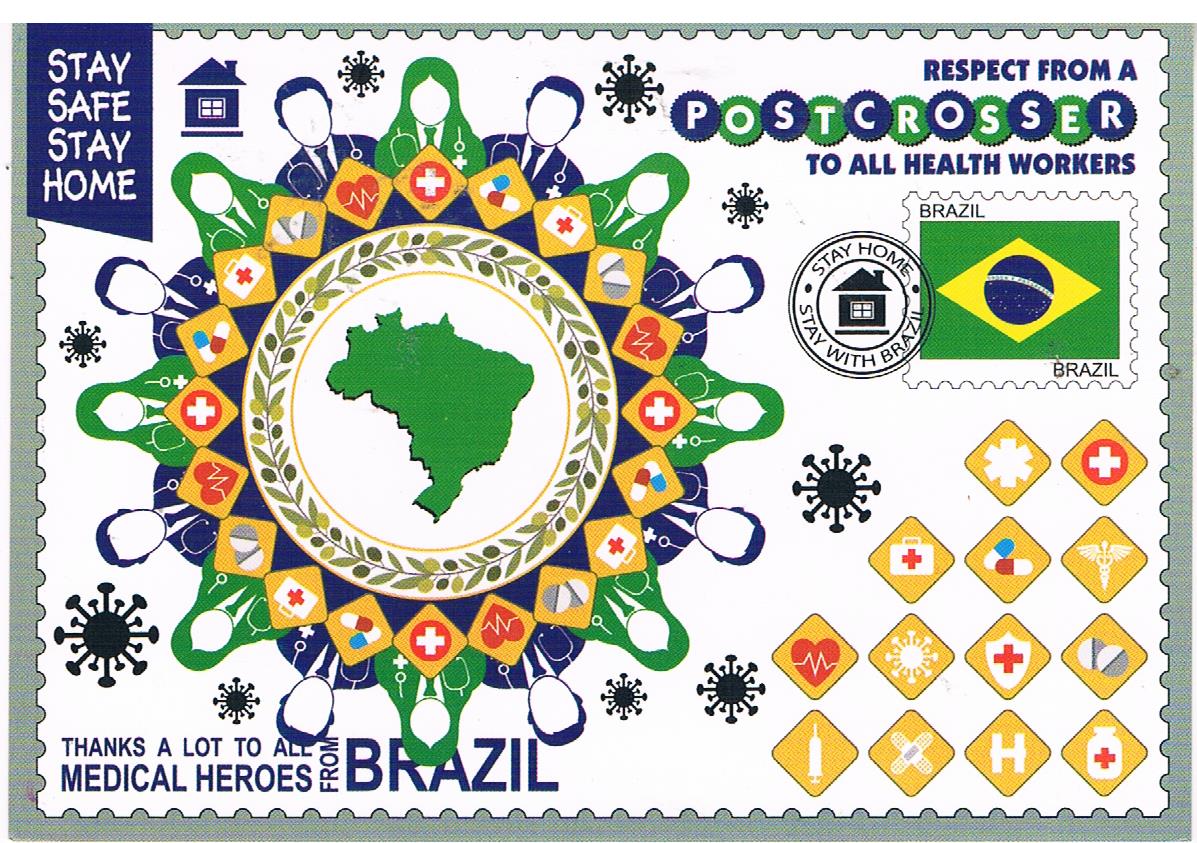The image is a thank-you card designed to resemble a postage stamp, predominantly featuring a green and yellow border and detailed imagery to honor medical heroes from Brazil. The card has a white rectangular center bordered with cut-out, curved half-circles, giving it the appearance of a perforated stamp. The upper left corner has a dark blue box with the text "Stay Safe, Stay Home," accompanied by a cartoon home icon in blue. The card has various lines of text, including "Thanks a lot to all medical heroes from Brazil" in the lower left corner, and “Respect from a Post Crosser to all health workers” in white letters within alternating blue and green circles on the right side.

The central design features a white circle containing a green map of Brazil, encircled by a leafy design. Surrounding this are alternating headshots of male and female doctors in blue and green, interspersed with gold squares containing icons like hearts, crosses, pills, and the COVID-19 virus symbol. Additional icons like the Caduceus, bandages, first aid symbols, and medical bottles in yellow diamonds are present in the outer ring. At the bottom right corner, the text “Respect from a Post Crosser to all health workers” is repeated, and below it are smaller images, including a stamp of the Brazilian flag and a circular logo with a home in the center, accompanied by the phrase “Stay Home, Stay with Brazil.” The imagery and text collectively convey gratitude and respect for medical workers battling the pandemic in Brazil.